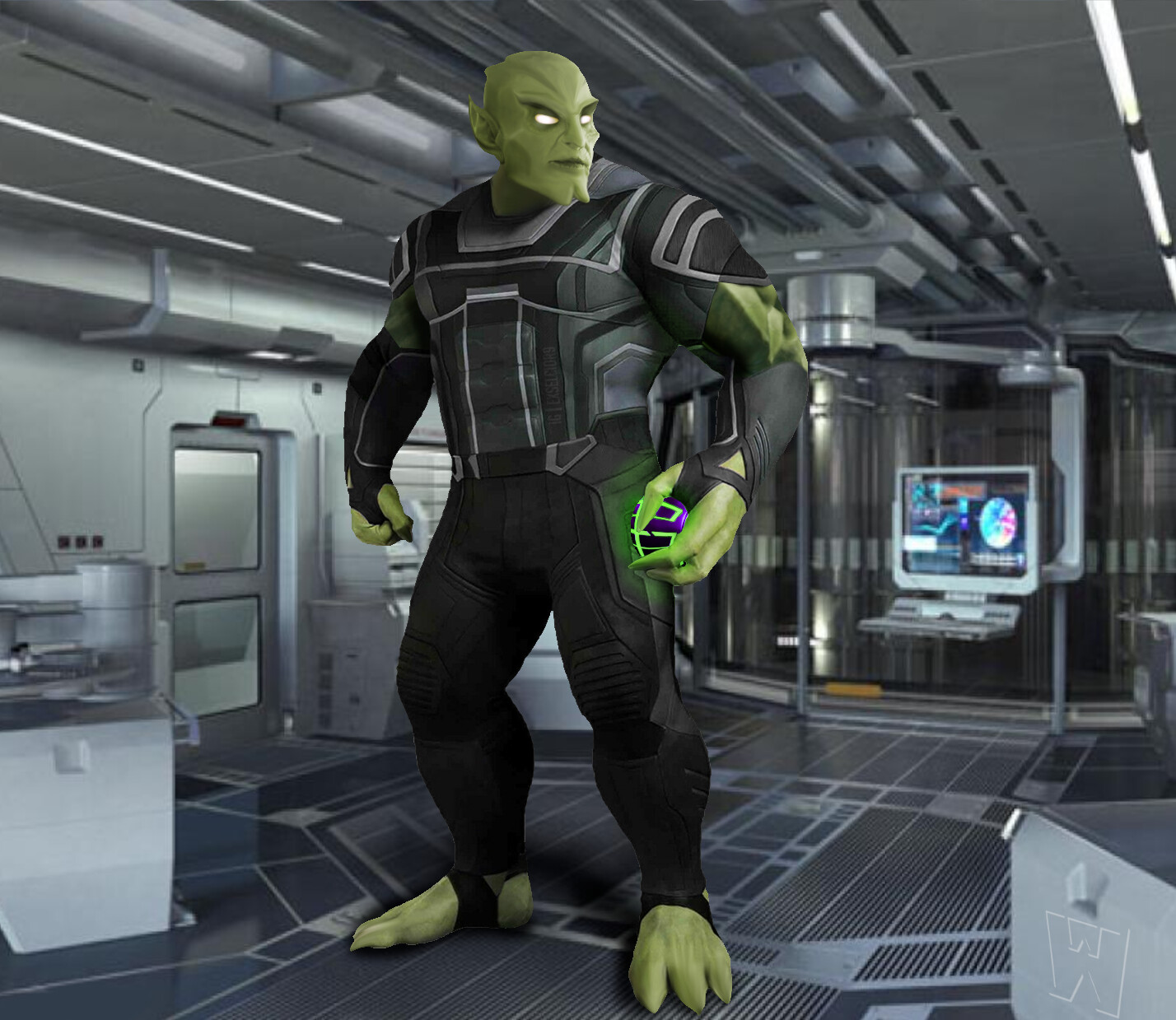The image portrays a large, green humanoid character that resembles a cross between the Incredible Hulk and an alien. He stands in the center of what appears to be a high-tech laboratory or futuristic facility, possibly even a spaceship. The environment is characterized by its metallic, gray steel interior, featuring various workbenches, thin horizontal lights, vented flooring, and a small, modern door. Behind him is a glass-enclosed area with a large computer screen displaying multicolored charts and a substantial keyboard setup. The green character has a distinctly muscular build, with prominent abs and broad shoulders accentuated by his tight-fitting black and gray suit. His face is fierce with pure white, slanted eyes, pointed ears, a ridged head, and a sharply angled chin. His hands and feet are green, with elongated fingers and claw-like toes. In his left hand, he holds a vibrant purple and neon green ball, emitting an ominous glow. His expression is alert and vigilant, as he gazes to the side, appearing ready for an imminent event.